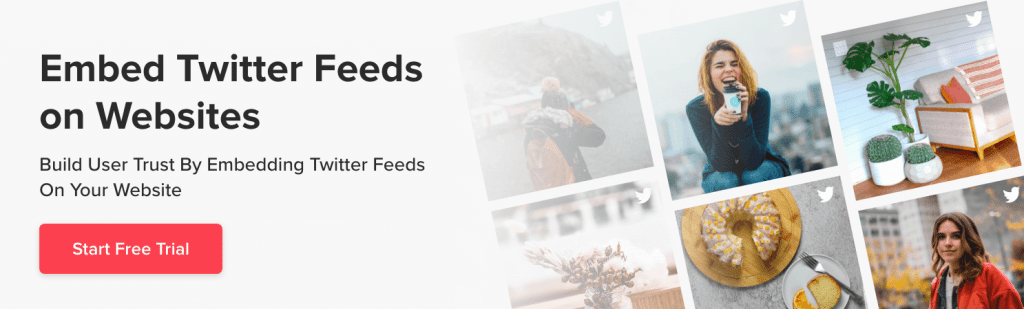This image, likely sourced from a website, has a rectangular green background and features a prominent rectangular red button in the lower left corner with bold white lettering that reads "Start Free Trial," indicating an online component. The upper left section of the image contains bold black text stating "Embed Twitter Feeds on Websites," with a smaller bold black subheading below that reads "Build user trust by embedding Twitter feeds on your website."

On the right-hand side of the image, there is a sequence of six square images, each angled slightly to the left. The top two images, shrouded in a light mist or fog, depict a person in a heavy jacket and backpack standing near water with a mountain in the distance. Below them, there is an indoor scene featuring a table with a vase of flowers. As the images progress towards the center, they become clearer. The top center image shows a woman smiling as she holds a cup of coffee near her lips, with a white Twitter bird logo in the upper right corner. Below this, there is an image of food on a cutting board, possibly a Bundt cake, also displaying the white Twitter bird logo.

The bottom two images depict a white couch with orange decor and three white pots with plants on the left side, again featuring the white Twitter bird logo in the upper right corner. The very last image shows a young woman wearing a red jacket, with long brown hair, standing in front of skyscrapers, with the white Twitter bird logo in the upper right corner again.

This detailed assemblage highlights the integration of Twitter feeds into a website, showcasing various scenarios, both indoors and outdoors, to emphasize user engagement and trust-building.